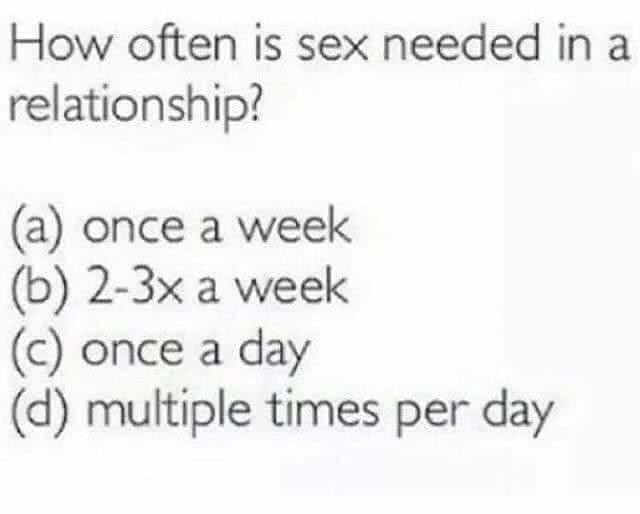The image displays a slightly blurry, typed question in a simple, Comic Sans-like font against a white background, seemingly part of a questionnaire. The question asks, "How often is sex needed in a relationship?" Below the question, there are four answer options listed vertically with two line spaces between the question and the options. Each answer is preceded by a lowercase letter in parentheses: (a) once a week, (b) 2-3 times a week, (c) once a day, and (d) multiple times per day. The numbers are formatted as "2-3" and "3x" for clarity. The layout suggests the text was printed and then photographed.